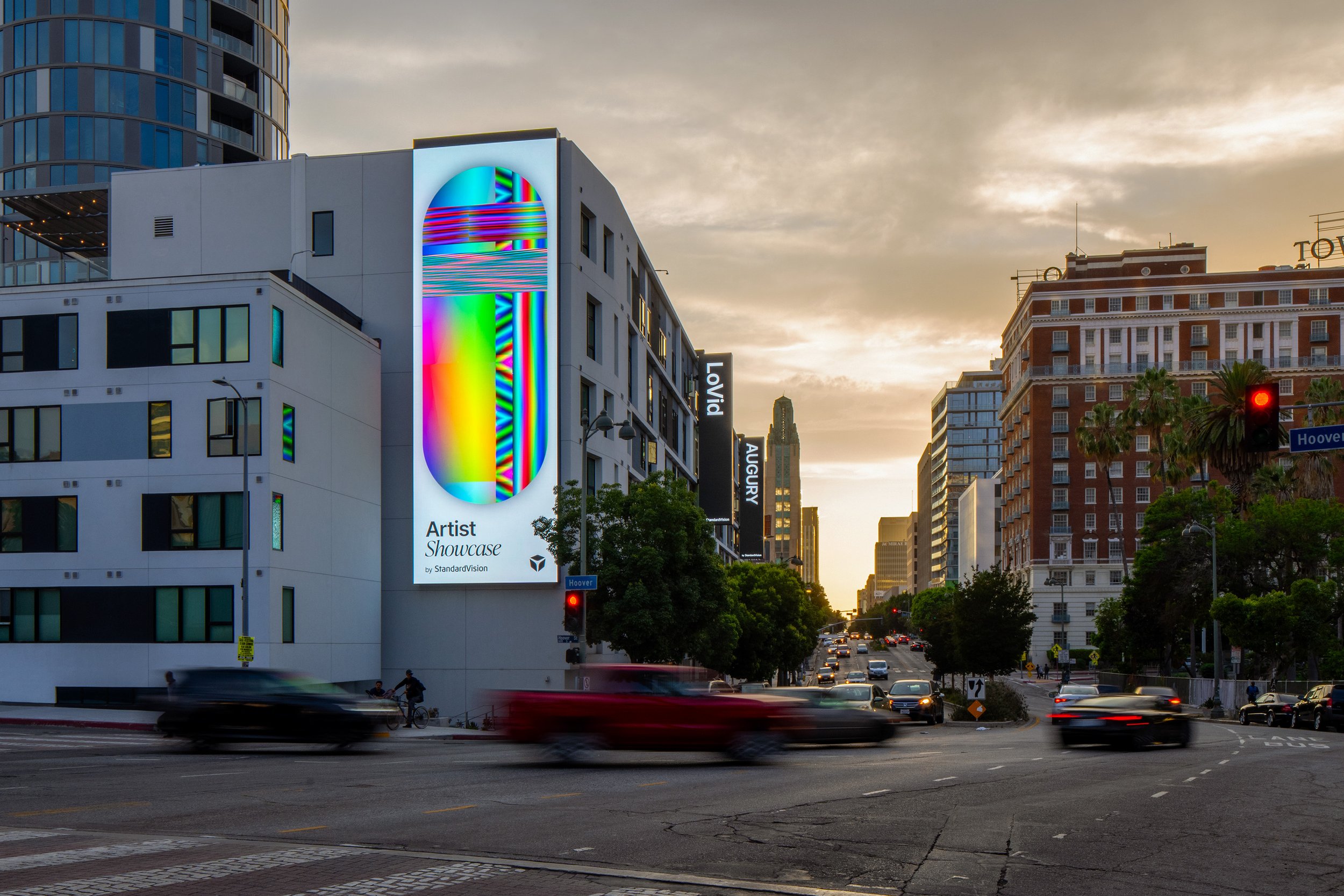The image captures a bustling cityscape during golden hour, with the natural light dimming under a cover of large, wispy gray clouds. In the foreground, several cars are blurred, whooshing past a traffic-light showing red. The street they occupy stretches into the middle ground, where it's lined with various apartment buildings. On the left, a modern, light-gray building, characterized by its square, contemporary design, features a tall vertical LED billboard. This billboard displays a vibrant, neon-colored artwork with geometric designs, highlighting an "Artist Showcase" by Standard Vision. Adjacent to this, other signs reading "LoVid" and "Ogri" are visible, attached to different apartment buildings that vary from four to six stories tall, while larger structures rise in the distant background. The building on the right contrasts with an older, dark-orange facade dotted with numerous windows, adding to the architectural diversity of the scene.